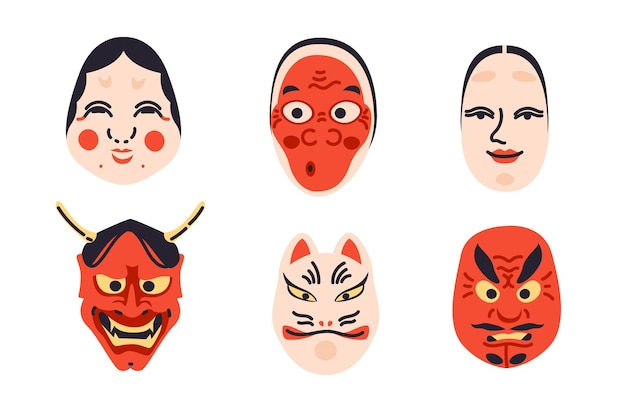The image is of six cartoonish, drawn faces arranged in a 3x2 grid with no background or border. The top row features three distinct characters: on the left, a lady with chubby cheeks adorned with round orange circles and a simple half-circle nose with two dots for nostrils; in the middle, a fully orange face with a bizarre sideways circular mouth expression; and on the right, a lady with red lips who is simply smiling. The bottom row illustrates more intense characters: on the left and right, two red-faced, angry-looking demons with exaggerated, wrinkled expressions and bared teeth; in the middle, a cream-faced, cat-like character with a devious look. Each face has exaggerated features, contributing to their unique and expressive appearances.